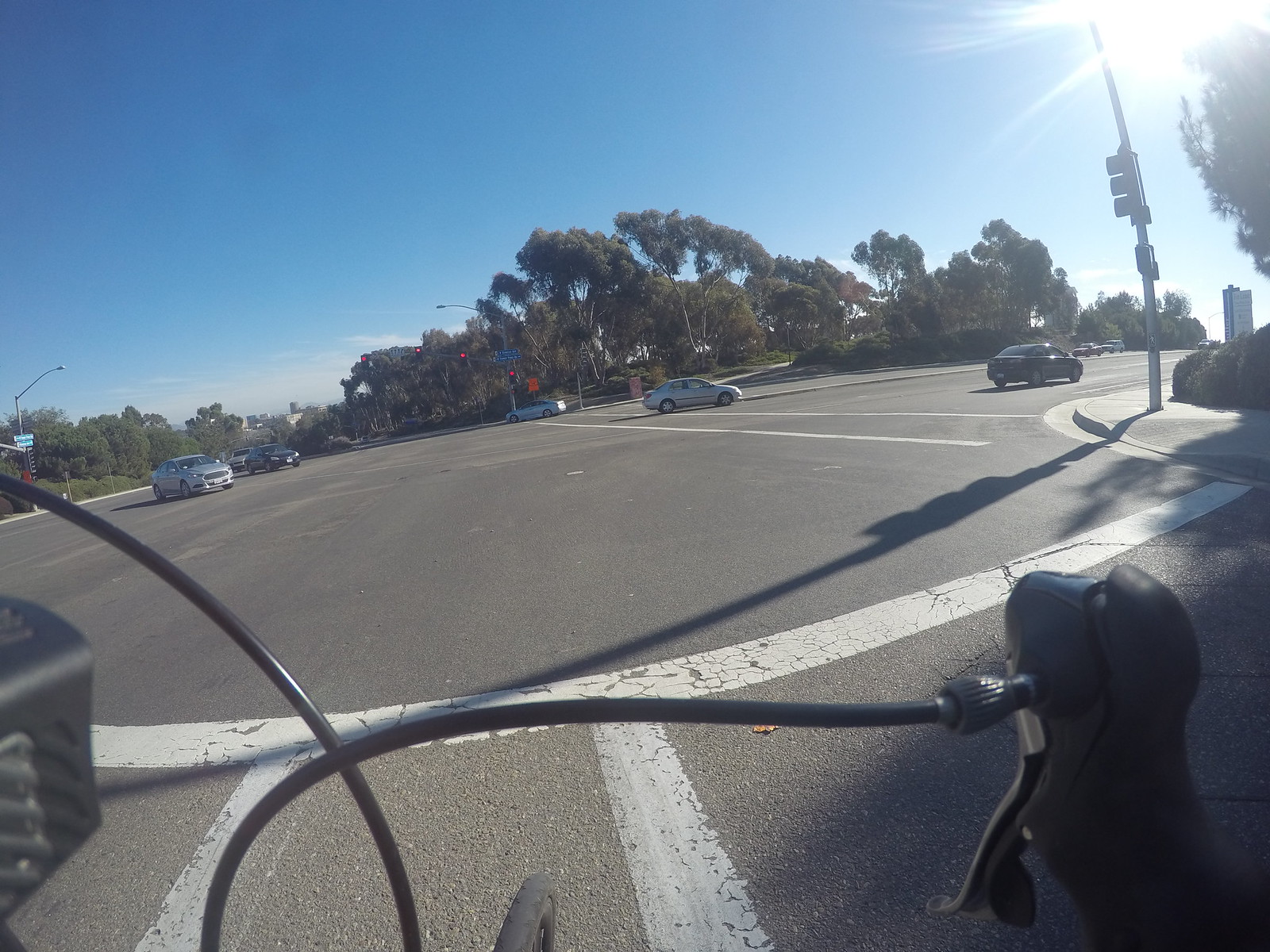This outdoor photo appears to have been taken by someone on a bicycle at a road intersection. Prominently in the foreground are the bicycle's handlebars, brake lines, and a front wheel reflector. A white crosswalk is painted on the black concrete ground just ahead. To the right of the frame, a traffic light stands upright on a metal pole, its red light illuminated. The street extends beyond the intersection, with multiple cars turning and blue street signs in view, though their text is unreadable. A grove of green-leaved trees with brown branches spans the background, suggesting a nearby park. The sky overhead is vivid blue and largely clear, with bright sunlight and rays visible at the top right. Overall, the scene is characterized by its bright, sunny day and active street setting.